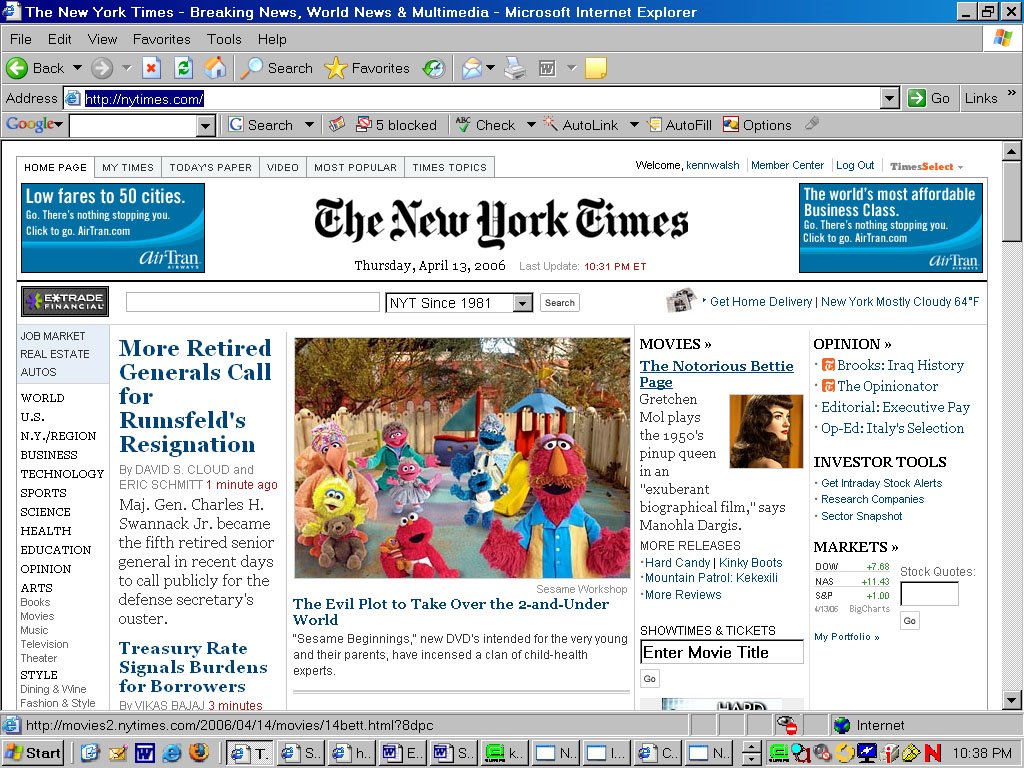A dated screenshot captures a New York Times webpage from an antiquated version of Internet Explorer. The date displayed prominently on the page is Thursday, April 13, 2006, perfectly aligning with the browser's archaic appearance. The interface is reminiscent of a physical newspaper, with the New York Times logo flanked by advertisements in the top right and left corners. 

The webpage is divided into sections visible on the side, presenting a typical layout of the time. Among the featured headlines are: "More Retired Generals Call for Rumsfeld's Resignation," "Treasury Rates Signal Burdens for Borrowers," "The Evil Plot to Take Over the To and Underworld," "Sesame Beginnings: New DVDs Intended for the Very Young and Their Parents Have Incensed a Clan of Child Health Experts," "Movies: The Notorious Betty Page," "Books: Iraq History," "The Opinionator," and a series on Executive Pay, both in editorial and op-ed formats.

This snapshot evokes nostalgia for the early 2000s internet era, where discussions such as executive pay, a topic still relevant today, were actively debated.